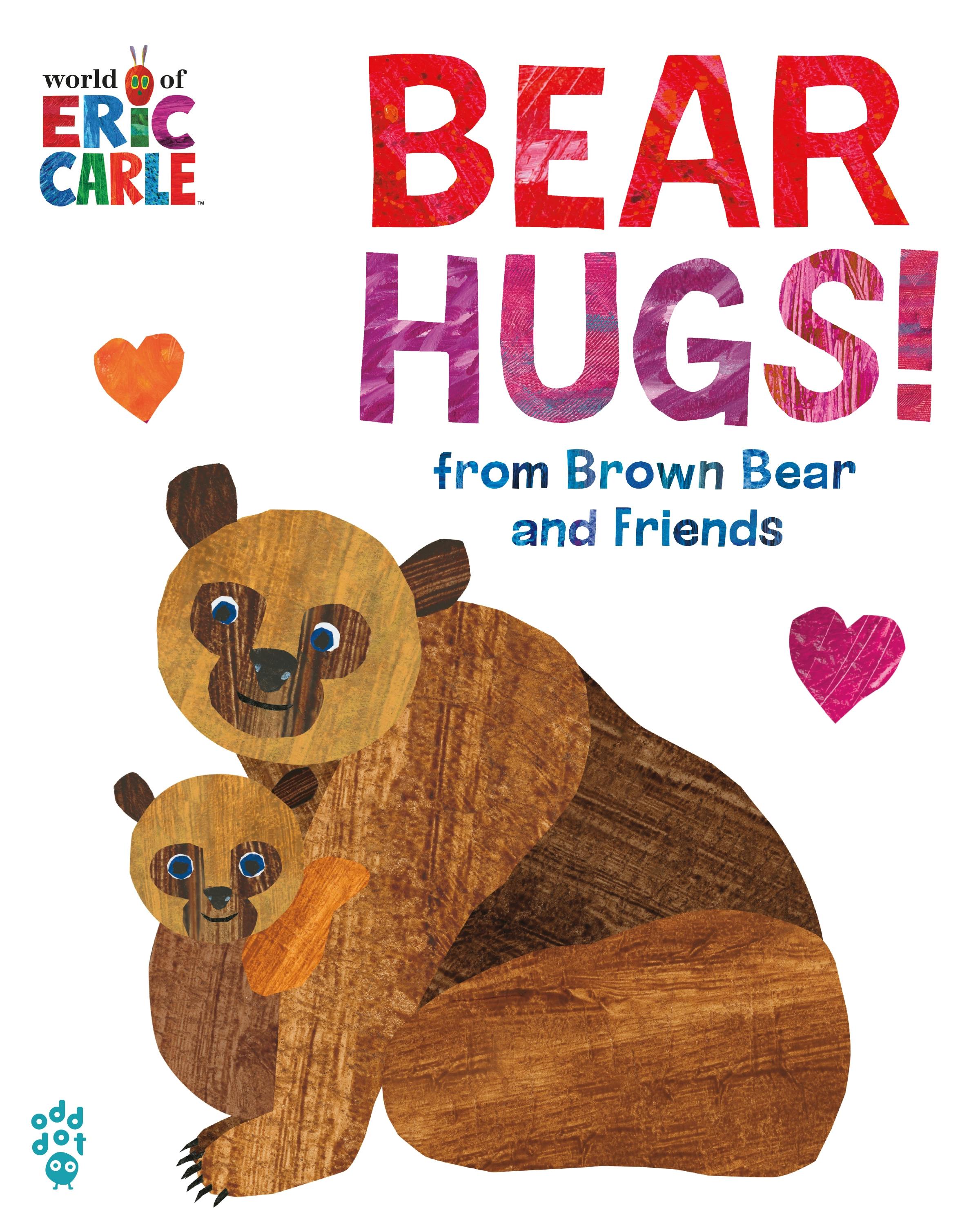This image features the front cover of "Bear Hugs! From Brown Bear and Friends," a children's book by Eric Carle. The top of the white cover reads "World of Eric Carle," with each letter in a different color, and a caterpillar forming the dot in the "i" of Eric. The title "Bear Hugs!" is in big, bold letters with "Bear" written in red and "Hugs" in purple, followed by an exclamation point. Beneath the title, it states "from Brown Bear and Friends." Dominating the cover is an illustration of two bears: a larger one, possibly a parent, sitting with its paws on the floor, dark brown ears, a light brown face, and darker brown mask around its nose, eyes, and mouth. The bear is smiling warmly. Clinging to it is a smaller bear cub, featuring the same happy expression, big round eyes, and tiny ears, both gazing forward. There are two hearts on the cover and, in the lower left corner, the small print "odd dot" along with a round circle and two eyes peeking out. The unique style of coloring and design adds to the charm of this book cover.